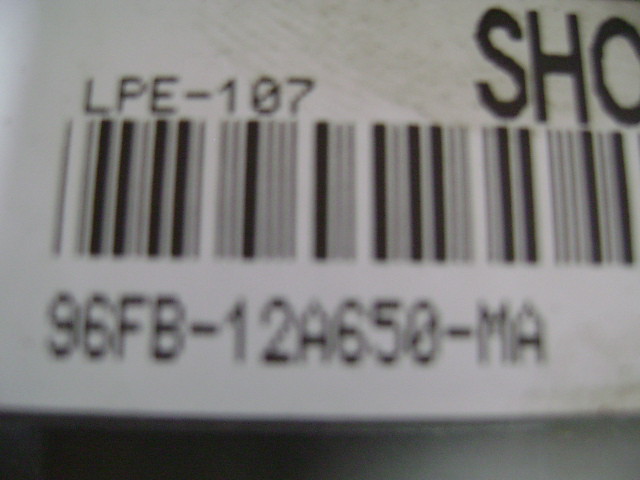This image features an extreme close-up of a barcode on the back of a product, likely medication. The photograph focuses tightly on the barcode, revealing partial details of the surrounding area. The alphanumeric codes accompanying the barcode are visible, displaying "LPE-107" above the barcode and "96FB-12A650-MA" below it. Due to the close proximity of the shot, the product itself remains unidentified.